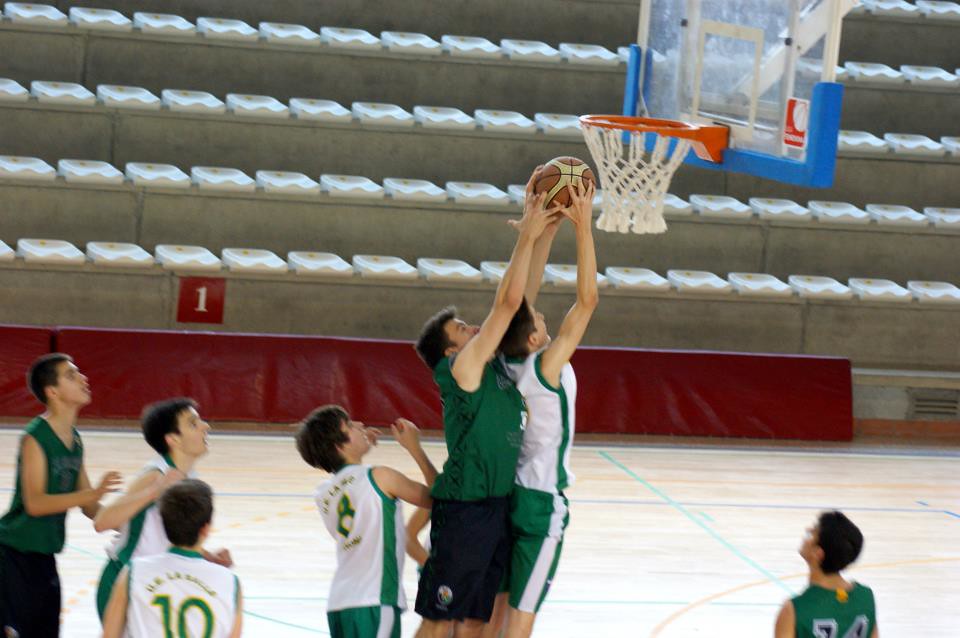In this dynamic indoor gym photo, two boys are the focal point as they leap into the air in an intense basketball face-off. The player in the foreground, closer to the right, is attired in a white uniform with green stripes and matching green shorts with white accents. He is seemingly attempting a dunk but hasn't quite reached the hoop yet. Beside him, a player in a green uniform with black shorts is jumping up, likely trying to block the shot. Surrounding these two are additional players: three teammates of the shooter, also in white and green uniforms, sporting numbers 8, 10, and an obscured number, as well as two more players in green uniforms, one of whom bears the number 14. They all appear to be partaking in or observing the action. The gym's background features slightly out-of-focus, manila-colored bleachers with maroon accents, suggesting a practice scrimmage or an informal game rather than an official match, as no referee is present. The atmosphere is charged with anticipation as everyone in the frame is eager to see the outcome of this crucial basketball play.